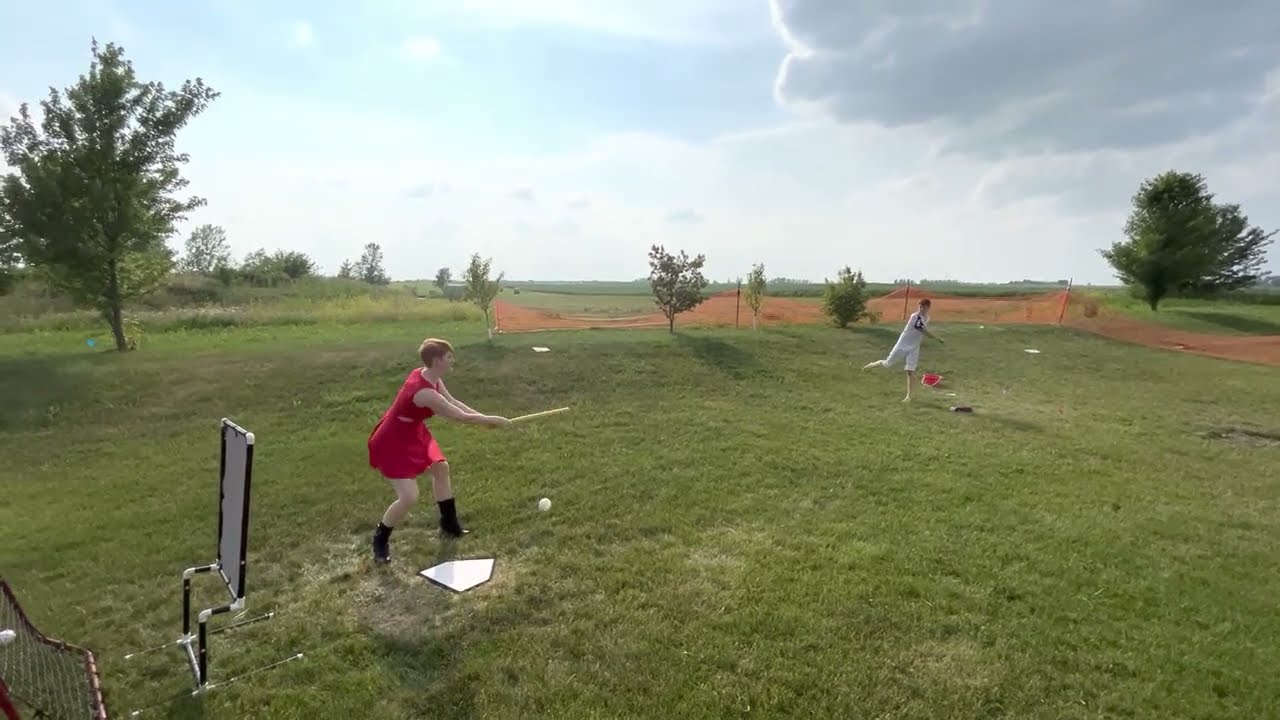In this outdoor daytime scene captured under a blue sky dotted with gray clouds, two individuals are engaged in a sporting activity on a large green grassy field. A man dressed in white shorts and a white shirt appears to have just pitched a white ball toward a woman. The woman, with short blonde hair, is swinging a small bat and is positioned at a white base plate typical of baseball settings. She is donned in a striking red dress and black stilettos. The white ball is seen slightly to the right of her bat, indicating she may have missed the swing. Behind her stands a net, possibly to catch stray balls. There is an orange net further off in the distance, blocking part of the field which transitions into a clay dirt area. The scene is framed by several trees; a large tree to the left, another significant tree in the back right-hand corner, and a collection of smaller trees dotting the periphery.